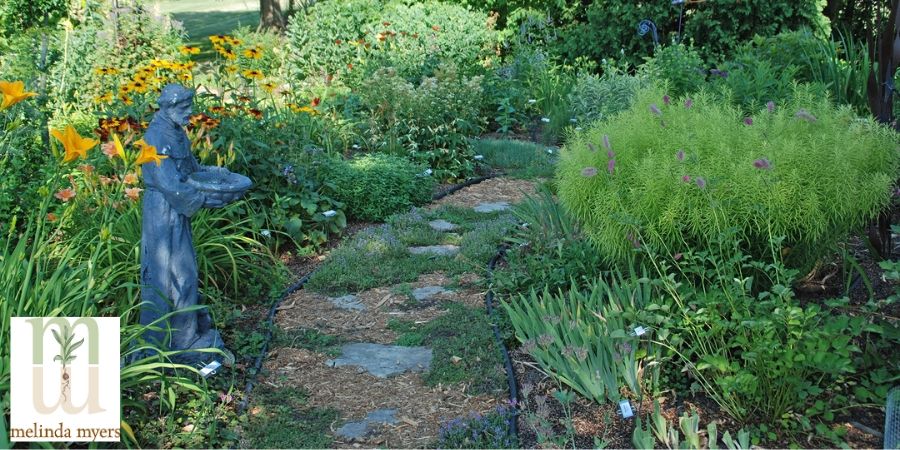This photograph captures a vibrant outdoor garden bathed in daylight, showcasing a meandering pathway lined with stones and bordered by rubber tubing. The path is a mix of small flat pavers and mulch interspersed with scattered green grass. To the left, a prominent figurine of a monk or possibly a saint, in long robes and with a tonsured hairstyle, holds a bowl that may serve as a birdbath. The garden is abundant with diverse flora, featuring yellow flowers like daisies or sunflowers, and purple blooms resembling lavender. Emphasizing the sunny, welcoming atmosphere, the bottom left corner of the image is marked with the logo and name "Melinda Myers," with the logo featuring two M's—one green and one tan—depicting the cycles of plant growth, with green leaves above and roots below.